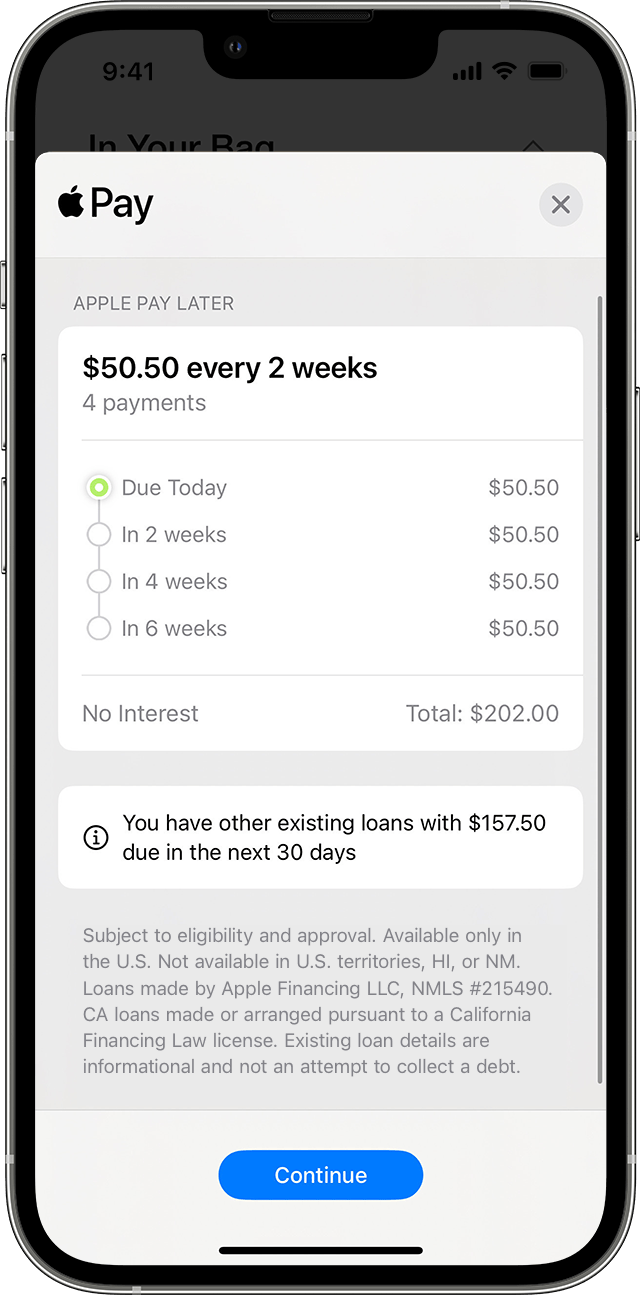The image features an Apple Pay interface displaying information about the Apple Pay Later service. At the top, the Apple logo is prominently displayed with the word "PAY" underneath. In the top right corner, there is an "X" icon for closing the interface. Below that, the header reads "Apple Pay Later."

A white rectangular box in the center of the image outlines the payment plan: "$5.50 every two weeks" across four payments. A gray line separates this section from the detailed payment schedule below, which states the following:

- Due today: $50.50
- In two weeks: $50.50
- In four weeks: $50.50
- In six weeks: $50.50

The total cost, with no interest, is displayed as $202.00.

Further down, there is another box containing a circled lowercase "i" for information. This section informs the user that they have other existing loans amounting to $157.50 due in the next 30 days.

At the bottom of the image, there is fine print that outlines the terms and conditions: "Subject to eligibility and approval. Available only in the U.S.; not available in U.S. territories, Hawaii, or New Mexico. Loan made by Apple Finance LLC, NMLS number 215490. California loan made or arranged pursuant."